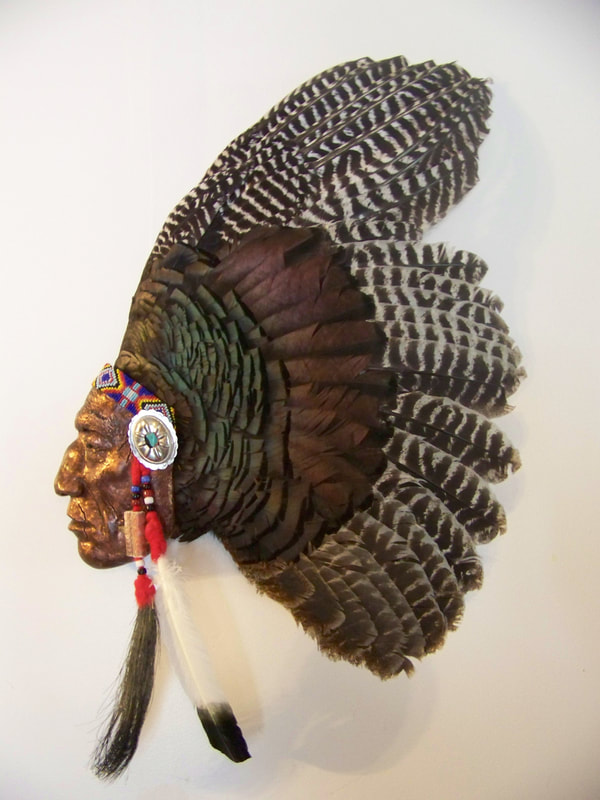The photograph showcases a detailed bronze sculpture of a Native American chief, portrayed in a left-facing profile against a tan background tinged with gray in the corners. The chief's weathered face, rich with character and creases, is adorned with a multicolored beaded headband. The headband features an intricate tribal design and bears a prominent turquoise medallion on the side, from which dangle red tassels ending in white feathers tipped with black. 

Attached to the headband is a majestic headdress, remarkably large—around four times the size of the chief's head—crafted primarily from turkey feathers. These feathers exhibit an array of colors: the ones closest to the head are a gradient of green blending to purplish brown, while the longer feathers at the back showcase striking black and white stripes, interspersed with shades of light and dark brown. Some feathers also display a mix of reddish-brown and golden hues.

Further enhancing the sculpture's vibrancy, beads in various colors—blue, red, white, yellow, orange, and black—are strung alongside the feathers. Overall, the headdress's feathers are meticulously layered, creating a visually captivating pattern that underscores the cultural significance and ornate beauty of Native American regalia.